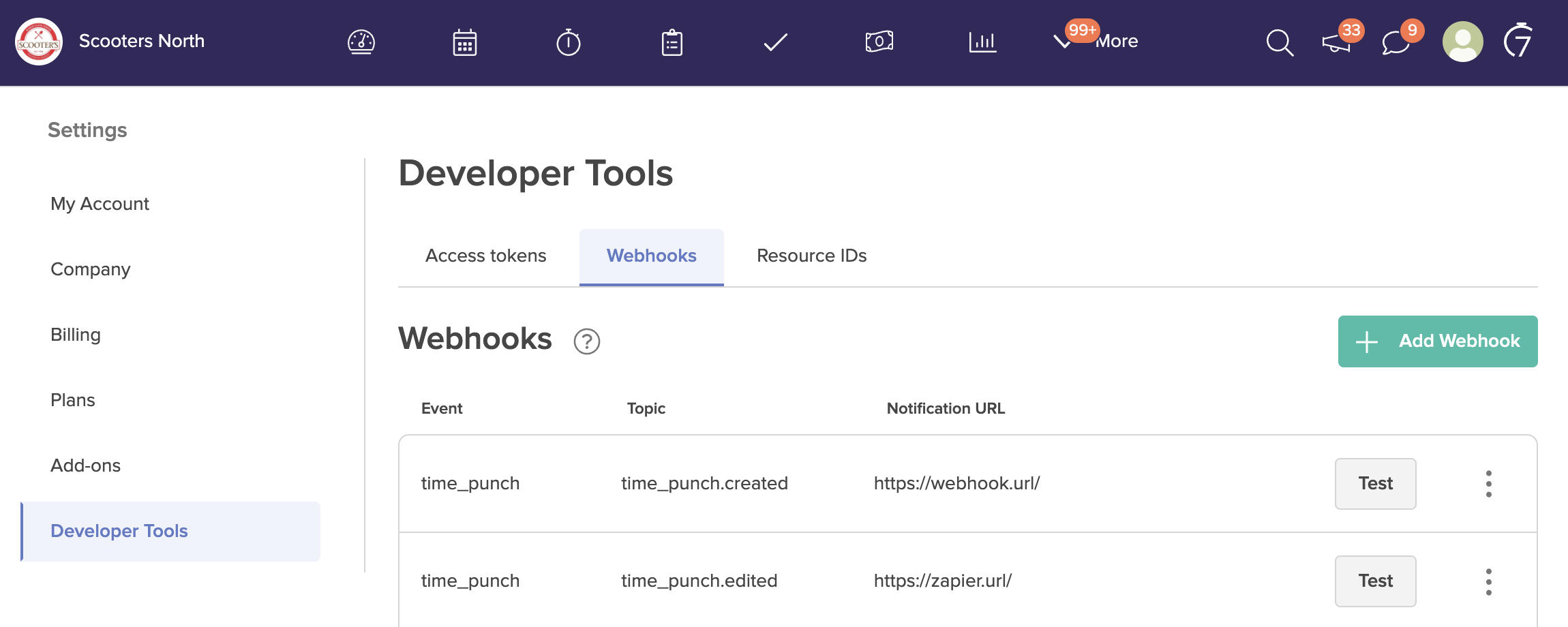The image appears to be a screenshot of a computer interface, likely part of an application or web-based management tool. The top border of the interface is blue. On the upper left corner, there’s a white circle with an orange inner circle containing the text "Scooters." To the right of this logo, the text "Scooters North" is displayed. A series of icons extends across the top of the screen, including a clock, calendar, stopwatch, clipboard, checkmark, graph, search icon, and text bubble. Additionally, there is a circle symbol featuring a generic person icon.

On the left side of the interface, a vertical menu bar is visible. The menu starts with "Settings" at the top, followed by options for "My Account," "Company," "Billing," "Plans," "Add-ons," and "Developer Tools." The "Developer Tools" option is highlighted in blue and written in blue font, indicating it is the active selection.

The right side of the interface has a white background labeled "Developer Tools" at the top. Beneath this heading, there are options for "Access Tokens," "Webhooks," and "Resource IDs." The "Webhooks" option is currently selected and is highlighted in blue. Under the "Webhooks" section, there is a circle with a question mark icon, followed by headings labeled "Event," "Topic," and "Notification URL," each corresponding to columns for listed items. Two entries are displayed in this list, both appearing to be related to time punches, and each entry includes a gray "Test" button to the right. Above this list and slightly to the right, there is a green "Add Webhook" button.